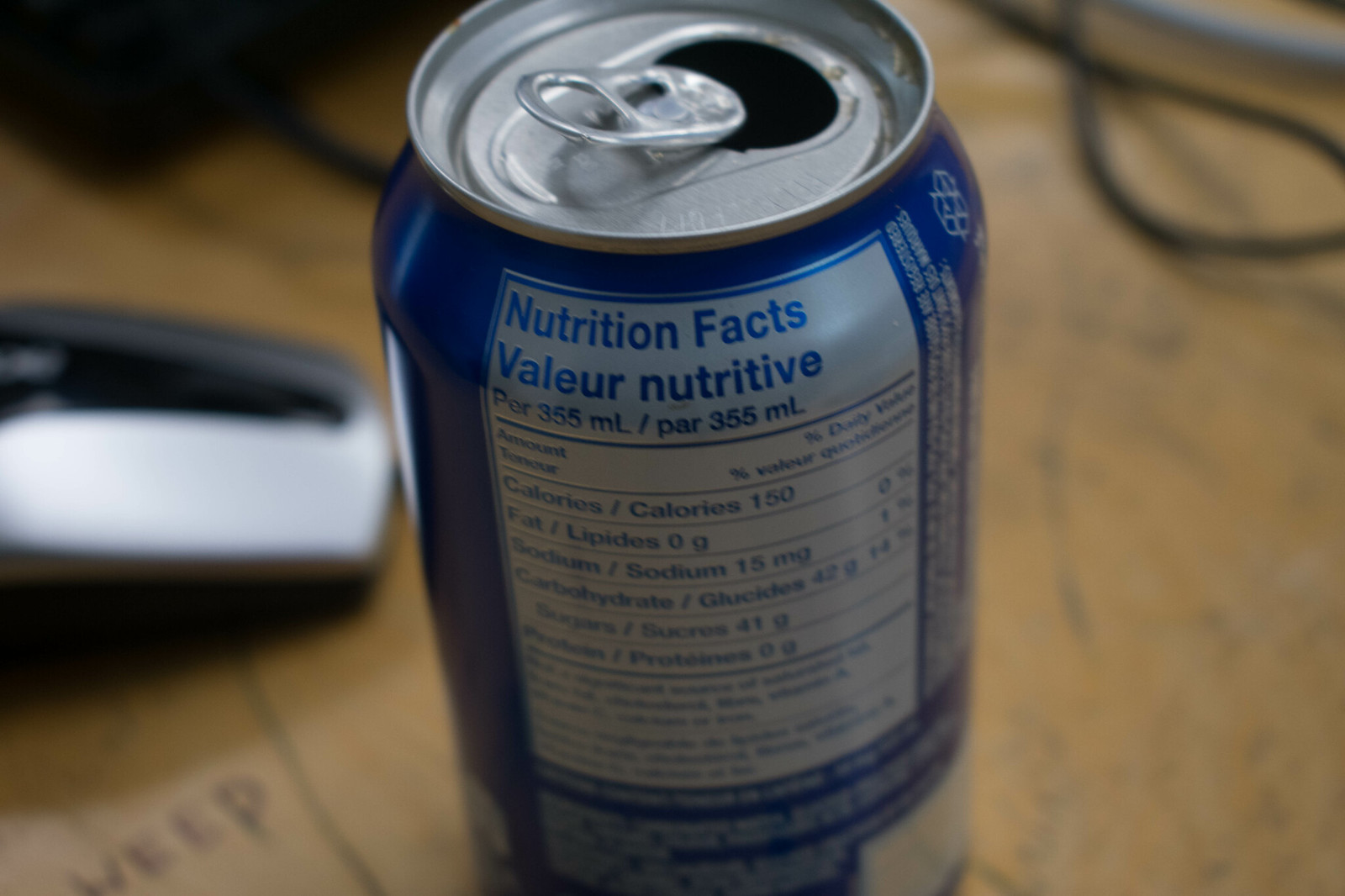This indoor color photograph features a blue soda can prominently displaying its nutritional information, both in English as “Nutritional Facts” and French as “Valeur Nutritive.” The detail reveals that the can holds 355 milliliters, containing 150 calories, 0 grams of fat, 15 milligrams of sodium, 42 grams of carbohydrates, and 41 grams of sugars. The can is positioned on a brown surface that has the word 'weep' written on it. Accompanying the can in the photograph is a silver object, and in the background, there is a black object with a black wire cord attached. The can itself has a combination of white background and both blue and silver lettering.